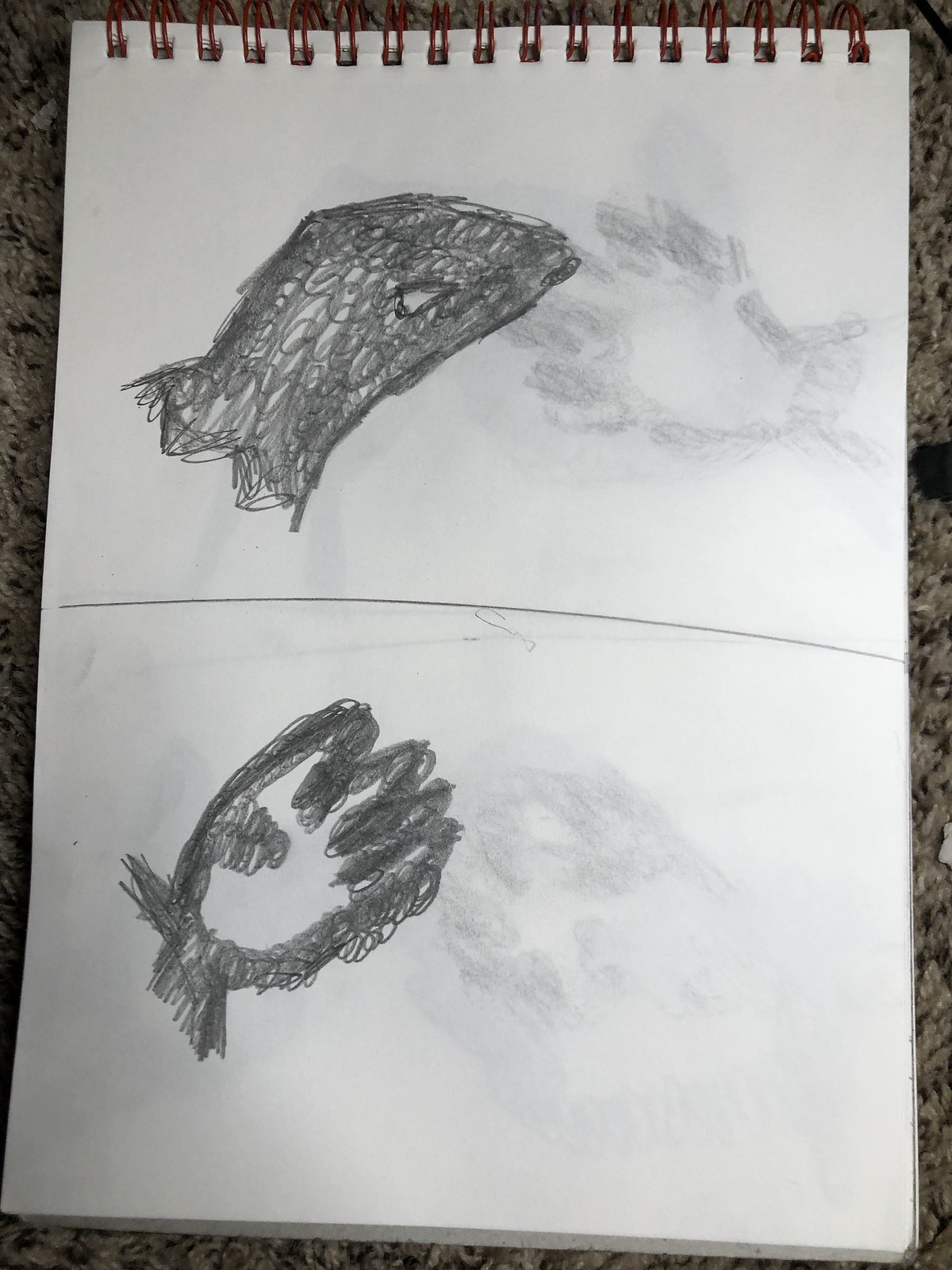In the vibrant photograph, a spiral-bound tablet sits on a pristine granite countertop, characterized by its white and gray hues with occasional dark splotches. The tablet is opened to a page adorned with various sketches. The spiral rings at the top possess a dark brown tint, securing the pages. Dominating the page is a central vertical line, splitting the paper into two distinct sections. 

On the upper part of the paper, a detailed sketch captures a hand forming a shadow-like creature, reminiscent of a bird's head, with carefully articulated curves. To the right, another hand sketch appears partially erased, offering a contrast between clarity and obscurity. Below these, a heavily bordered hand-like shape is filled with dense scribbles, adding a raw, expressive element to the page. The amalgamation of sketches provides a glimpse into the artist's creative process, all set against the naturalistic backdrop of the granite countertop.